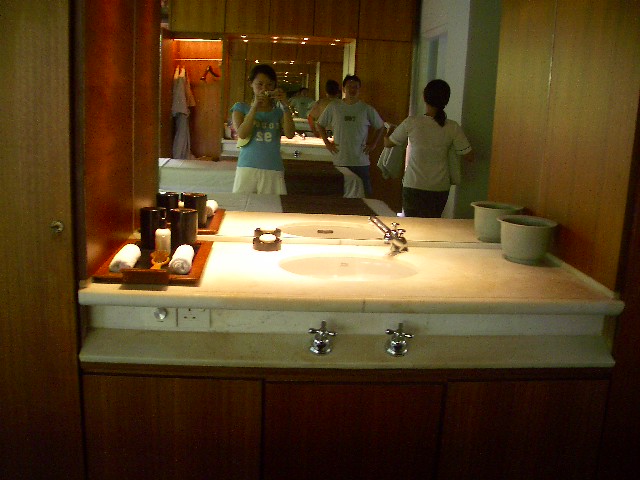In this photograph taken in a bathroom, three individuals are captured standing in front of a mirror, which creates a repetitive reflection effect. The woman on the left is wearing a blue t-shirt and white bottoms and is holding a camera to take a selfie. Next to her, a man in a gray t-shirt stands with his hands on his hips. On the far right, a woman with her back to the camera is clad in a white t-shirt and black bottoms, holding what appears to be towels or sheets. 

The bathroom sink counter is detailed with a wooden tray on the left side, adorned with black candles, white towels, and a bottle of lotion. There is also a black soap dish with a white bar of soap. On the right side of the counter is a flower pot. Below the sink, two large handles for the water are visible. To the side, a closet is seen reflected in the mirror, showing hanging clothes and hangers. The counter itself appears to be cream or tan in color, adding to the detailed and organized setting of this bathroom, which could very well be in a hotel room.